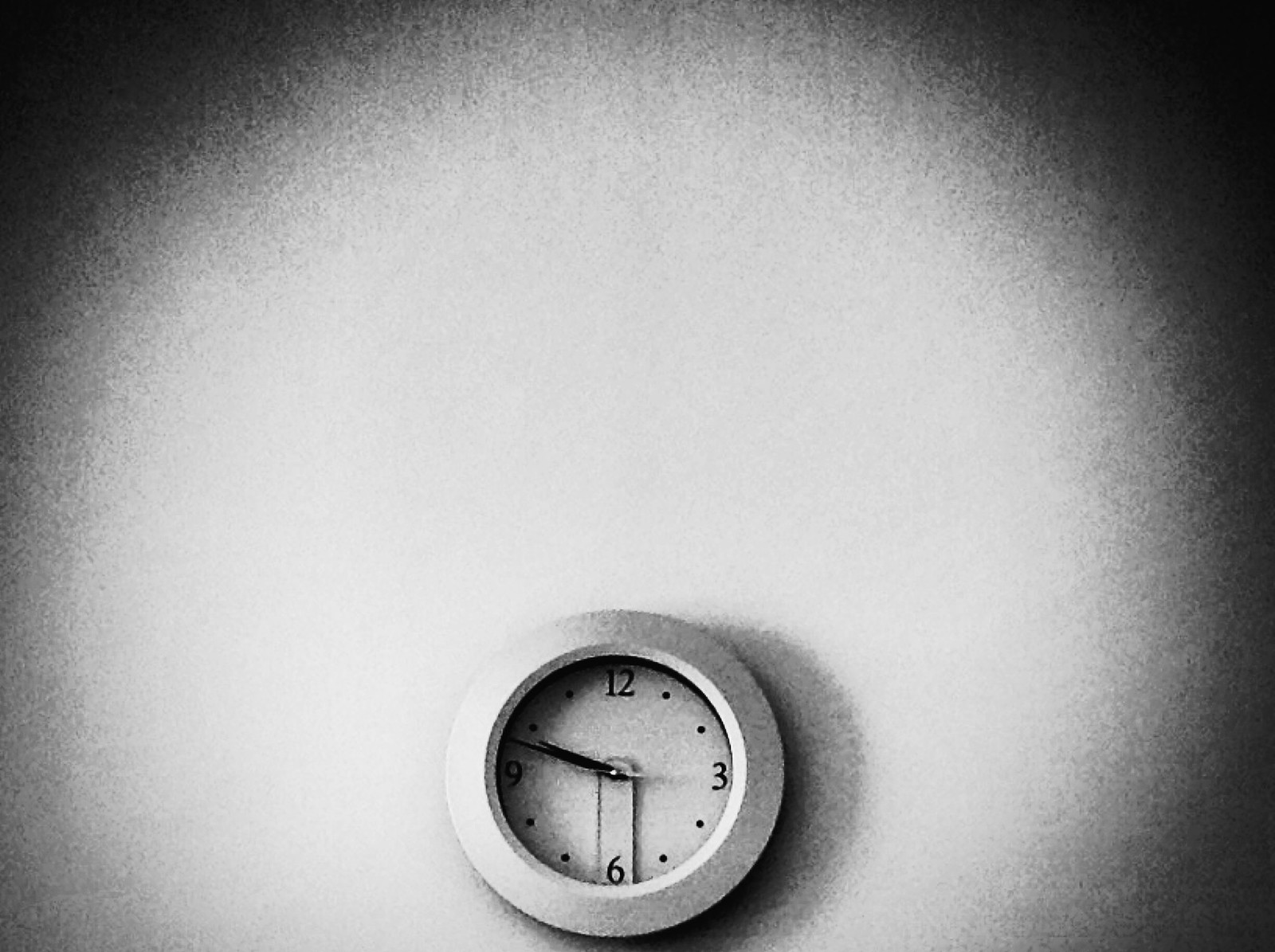In this black and white photograph, we observe a simple wall clock positioned near the bottom of the frame. The clock features a white border with a subtle indentation, lending a touch of elegance to its minimalist design. The clock face displays the numerals 12, 3, 6, and 9, while small dots mark the positions of the other hours. The minute hand is long and dark, contrasting with the shorter hour hand, and there is a barely discernible second hand that might be white. The clock is mounted on a white wall, contributing to the overall simplicity of the scene, although the graininess of the image adds a textured, vintage feel.